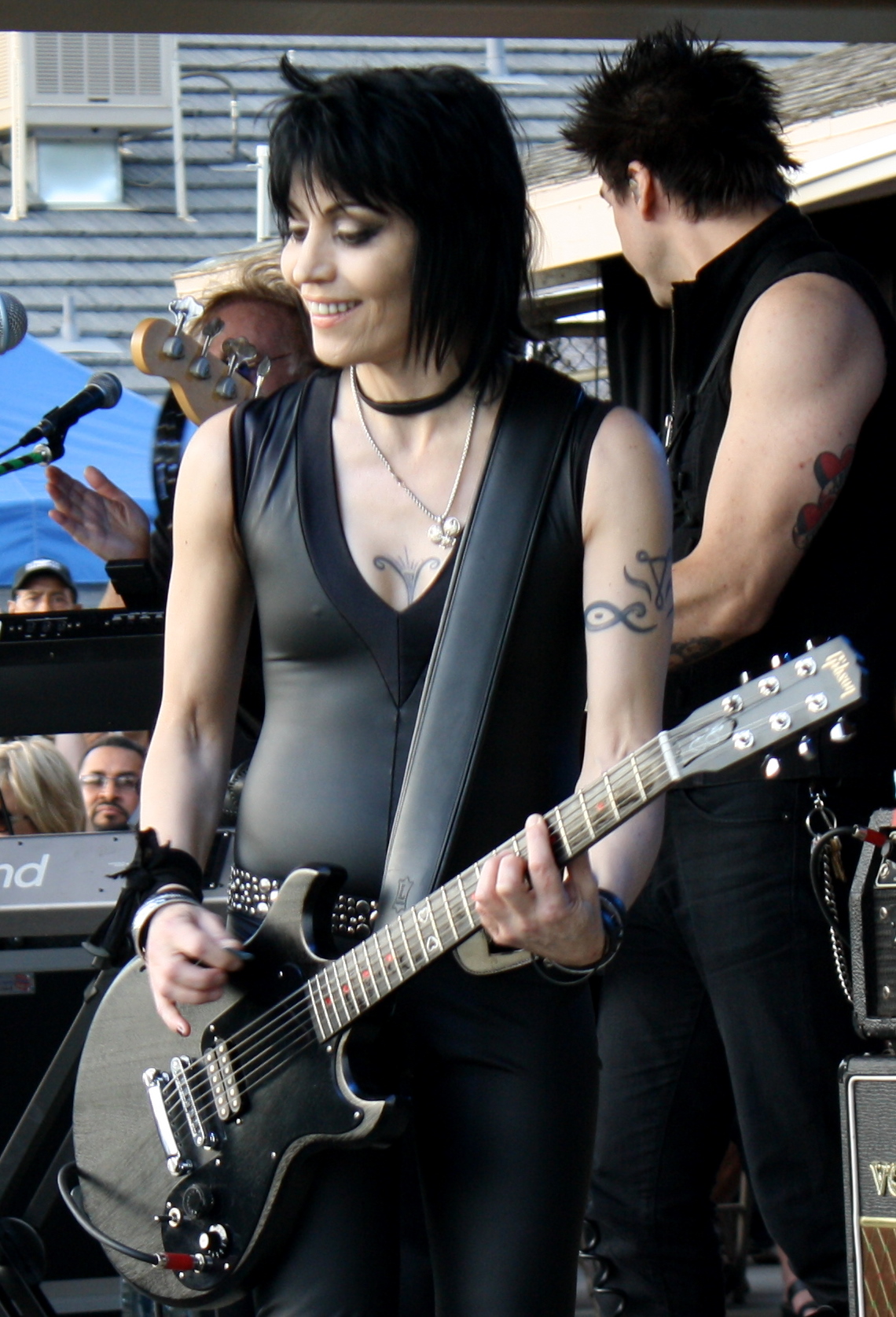This photograph captures Joan Jett in the midst of an energetic outdoor performance. Dressed in tight, form-fitting black leather pants and a v-neck leather tank top, Joan exudes rock stardom. Her outfit is accessorized with a studded belt and a delicate choker necklace. She has short, pitch-black hair, matching eyebrows, and lashes, and she accentuates her look with pink lipstick. Prominently visible are her tattoos: one below her neckline, resembling cleavage, and another on her left arm, depicting a triangular pattern with loops and a swirl. 

Joan is playing a black electric guitar, a chiseled smile on her face, holding the instrument with her left hand while strumming it with her right. The guitar is secured with a black strap featuring an "L" insignia. In the background, a male musician, clad in black jeans and a black jacket, likely playing a bass guitar, can be seen with his head turned away from the camera. Additional stage elements include a microphone on a stand, a Roland keyboard, and the edge of an amplifier and speaker system.

The setting is outdoors, evidenced by the distant shingled roof, roof-mounted air conditioner, vent pipes, yard light, and a blue tarp. Fans are gathered around the stage, intently watching Joan, creating an atmosphere of excitement and adoration.